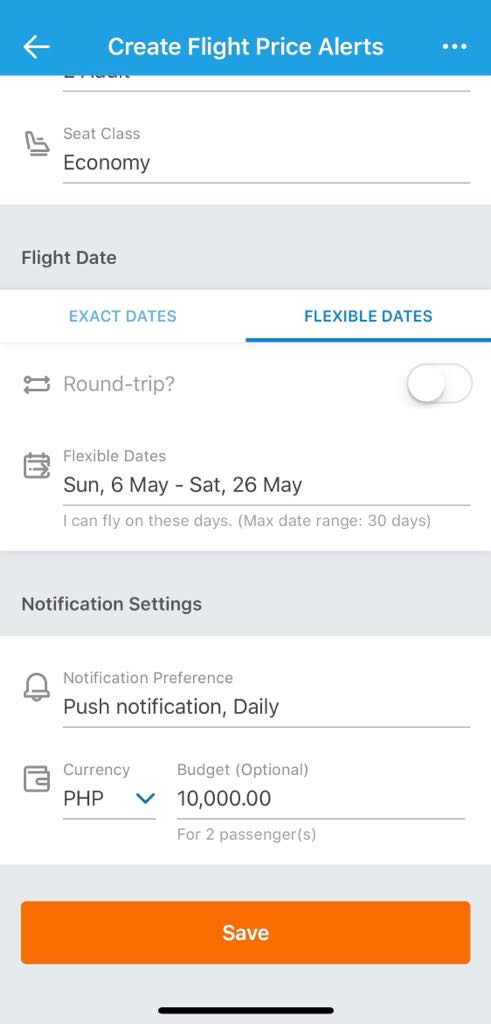This is a detailed screenshot from a flight booking website, showcasing a vertical display. At the top of the screenshot, there's a blue horizontal banner. On the left side of the banner, there's a left-facing white arrow, and next to it, the phrase "Create Flight Price Alerts" is printed in white. To the far right of the banner, two white dots are visible.

Below the blue banner, the background color shifts to white. Here, an icon representing a seat is displayed along with the text indicating the seat class, which is "Economy." Further down, a gray horizontal banner separates this section from the next one. Underneath the gray banner, there are several text entries. It starts with "Flight Date," followed by options for "Exact Dates," "Flexible Dates," and "Round Trip."

For "Flexible Dates," the text specifies the date range from Sunday, May 6 to Saturday, May 26, along with the note "I can fly on these days." Additionally, it's mentioned that the maximum date range allowed is 30 days. The notification settings indicate push notifications are set to be delivered daily.

The currency for the price alert is set to PHP (Philippine Peso). There's an optional budget field that is filled in with the amount $10,000 for two passengers.

At the bottom of the page, set within a gray rectangle, lies a smaller orange rectangle, centered and featuring the word "Save."